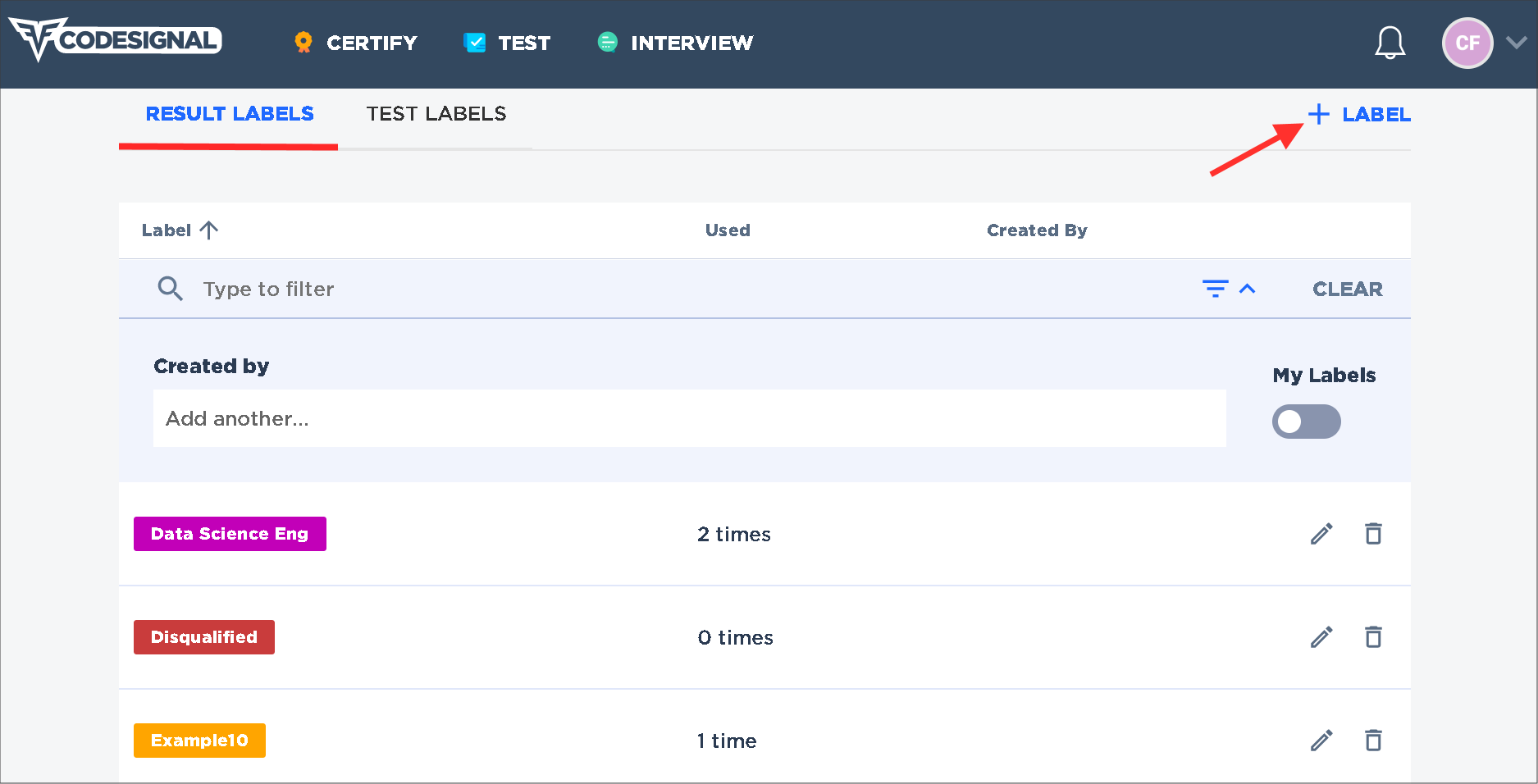This is the user interface for CodeSignal. On the extreme top-left corner of the page is the CodeSignal logo followed by three tabs labeled "Certify," "Test," and "Interview." On the top-right corner, there's a user avatar represented by a pink circle with the letters "CF." Below this black navigation bar, there are two additional tabs: "Result Labels" and "Test Labels." The "Result Labels" tab is highlighted with blue text and has a red underline. To the right of this tab is an "Add Label" function. Beneath this section is a table with three columns and a filter bar to sort the results. Within the table, the first column displays colored rectangles with white labels such as "Data Science N," "Disqualified," and "Example 10."